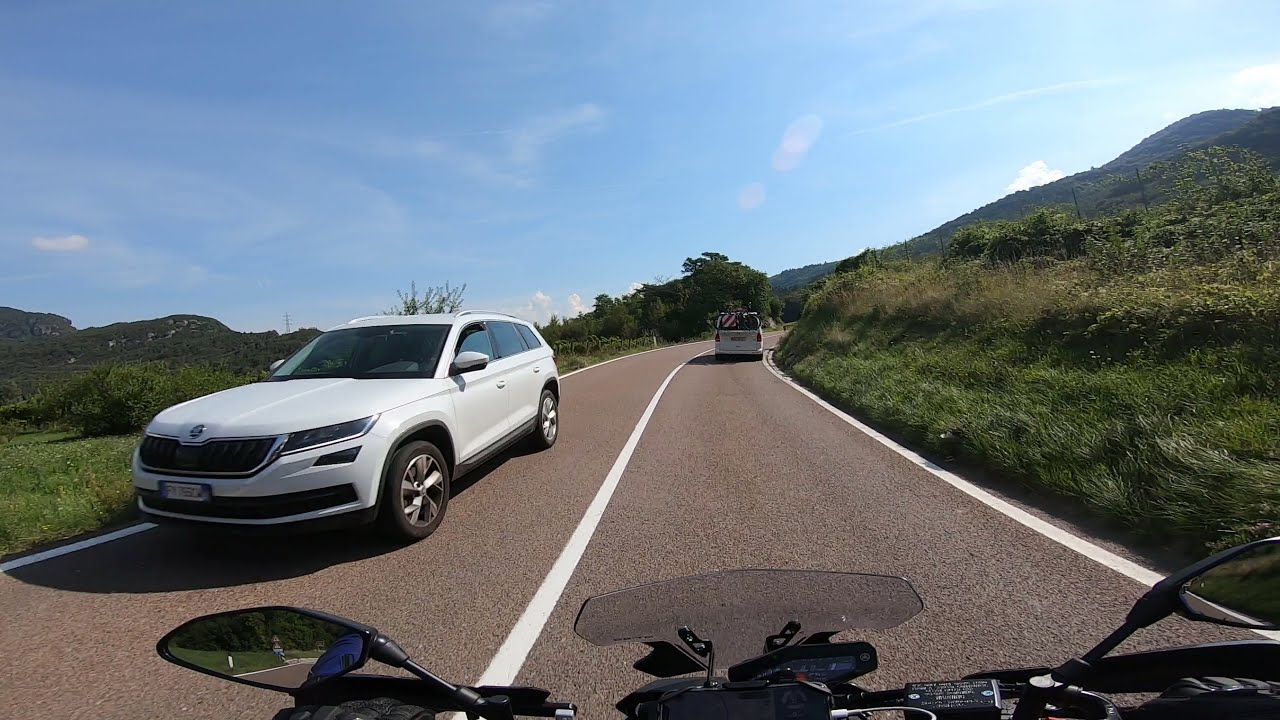The photograph captures the perspective of someone riding a motorcycle on a narrow, two-lane road. The motorcycle's handlebars and rearview mirrors are visible at the bottom of the frame, with the rider wearing gloves. The road, flanked by white lines on both sides and a solid white line in the middle, extends from the bottom of the frame up to the center before curving to the right around a grassy hill. A white van is directly ahead, while a white SUV with its driver’s window slightly rolled down is approaching from the opposite direction in the left lane. The landscape features lush green grass with shrubs and bushes on both sides of the road, a few scattered trees, another hill in the background to the right, and a serene blue sky overhead.